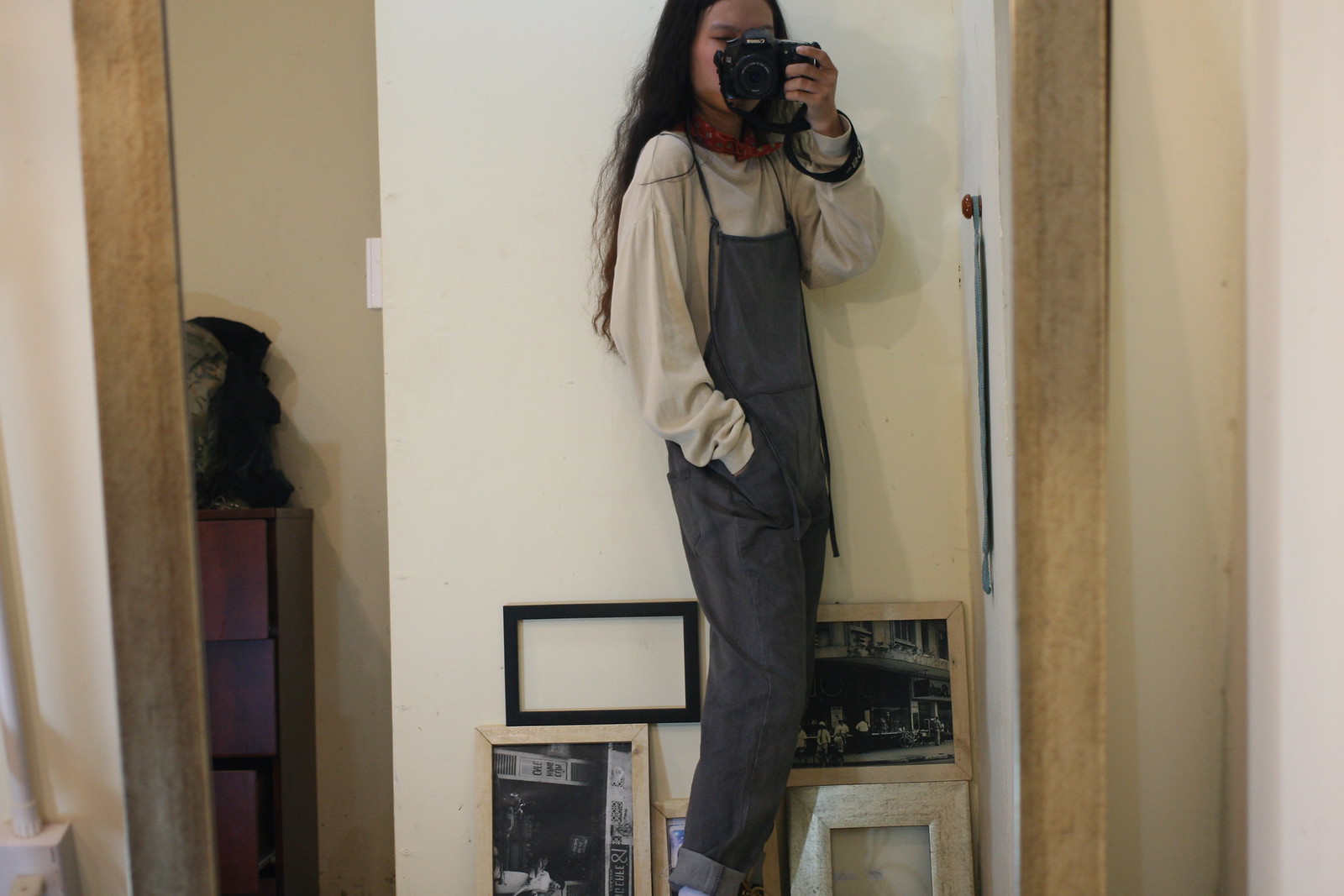A young Asian woman with long, wavy black hair is taking a selfie with a black camera, reflected in a mirror. She is wearing gray baggy overalls over a cream-colored long-sleeve shirt, and she has black bracelets on her wrist, which is holding the camera. The mirror is framed with medium to light brown natural wood and behind her, on the wall, you can see several picture frames. Three of the frames contain pictures, two of which are black and white, while the other two frames are empty. In the reflection, there is a white door or wall in the background and to the left, a dark brown-framed cabinet. The overall background features shades of gray and light gray.